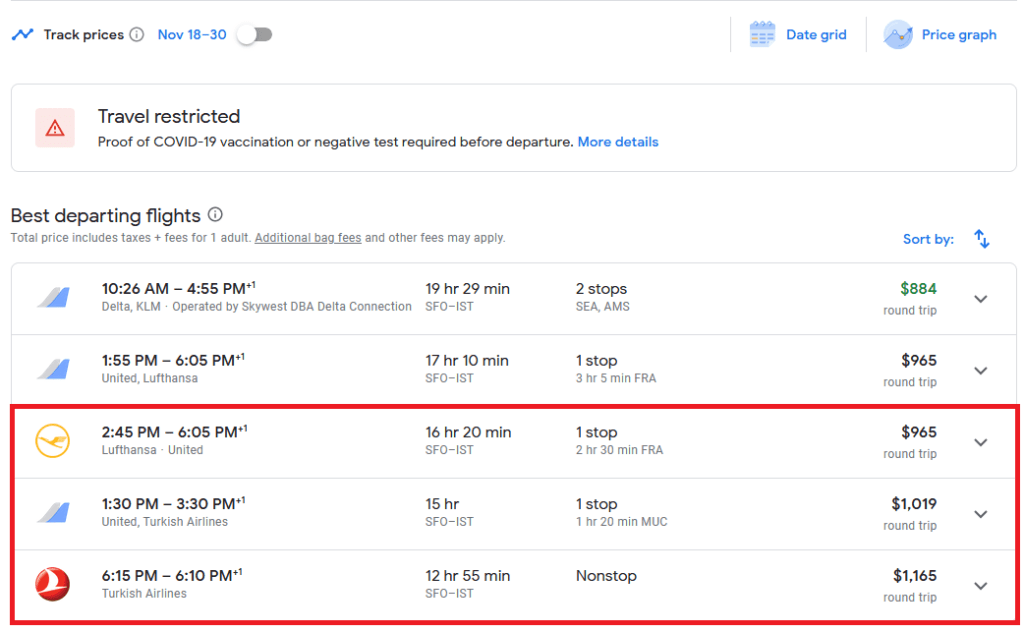This cropped screenshot of a Google Flights page is a comprehensive view of flight options and associated details for travel dates from November 18th to 30th. At the top left corner, the "Track prices" feature is visible but currently toggled off. To the right, "Date grid" and "Price graph" are hyperlinked in blue, offering alternative ways to view fare information.

An advisory banner is prominently displayed below, featuring a red box with a triangle and exclamation point, indicating important travel information. It highlights that travel is restricted and requires proof of COVID-19 vaccination or a negative test result before departure, with a "more details" link hyperlinked in blue for further information.

The section below the advisory banner is titled "Best departing flights," and notes that the total prices include taxes and fees for one adult, with a reminder that additional bag fees and other potential charges may apply. The additional bag fees link is hyperlinked for more information. On the far right, the "Sort by" option, accompanied by an up and down arrow icon, allows users to reorder the flight list displayed vertically on the page.

Three flights at the bottom of the list are highlighted with a red box, edited onto the screenshot to bring attention to these specific options. This detailed view assists users in understanding their travel options, associated costs, and necessary documentation for their journey.